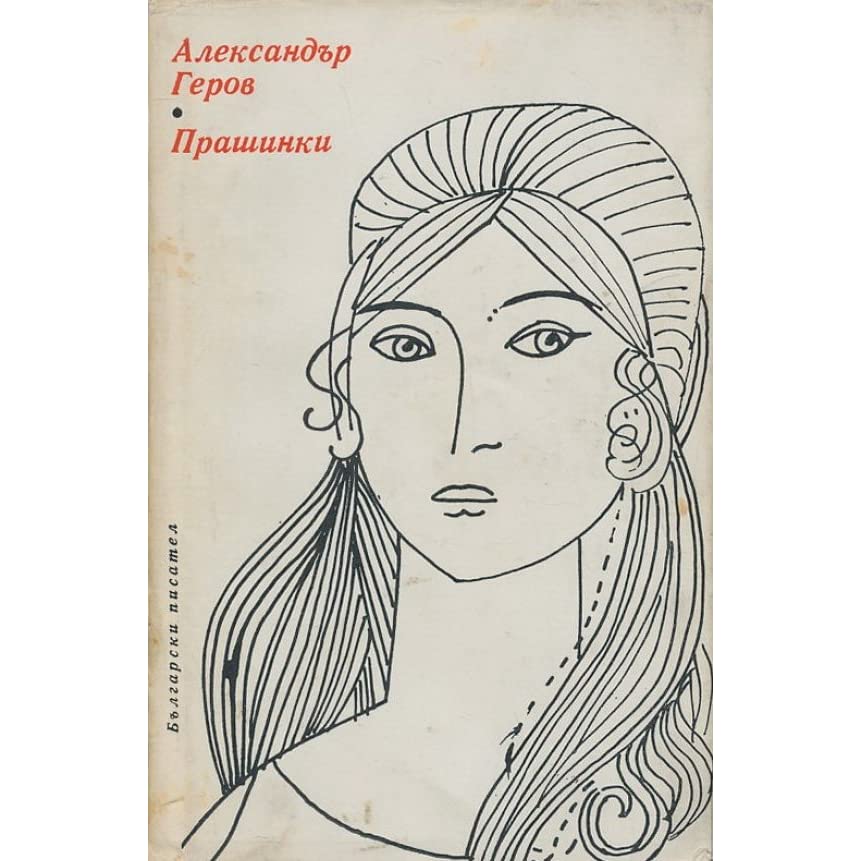The image is a meticulously drawn black and white sketch of a young woman on what seems to be a pamphlet or book cover. The drawing captures the woman's upper body, focusing on her face, neck, and the top of her chest. She has long hair styled in two side pigtails or ponytails, with bangs that crisscross over her face. Her eyes are large and expressive, gazing directly at the viewer, while her nose is depicted as somewhat flat at the end, without a distinct nose tip. No jewelry adorns her, and she appears to be wearing a simple dress. Above the portrait, there are words written in what is likely Russian or Cyrillic script, arranged in three lines. The text contains several recognizable characters but is otherwise unreadable. Notably, some of the text is also highlighted in orange with a black dot. The overall expression on the woman's face is serious, and the fine pencil linework gives the sketch a delicate yet detailed appearance.